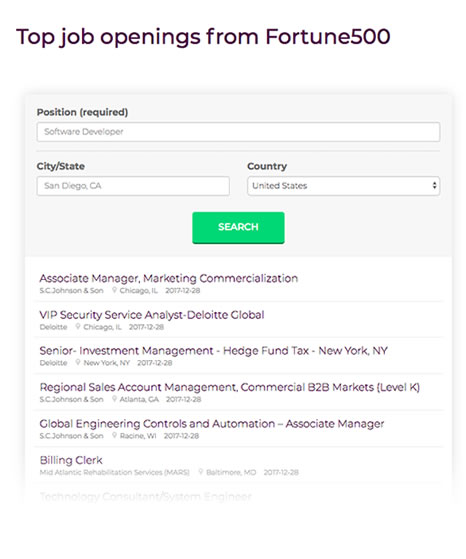This is a screenshot from a website featuring job listings titled "Top Job Openings from Fortune 500" at the very top in black text. The image showcases a user interface module with a 3D shadowed background. The module prominently displays a heading labeled "Position (required)" followed by a text box for entering the job position name. Below this, a line break separates two side-by-side dropdown boxes: the left one for "City/State" and the right one for "Country." A green "Search" button is centrally located beneath these dropdowns.

The job listings are displayed on a white background. They include:

1. **Associate Manager Marketing Commercialization**  
   - **Company:** SC Johnson & Son  
   - **Location:** Chicago, Illinois  
   - **Date:** 2017-12-28  

2. **VIP Security Service Analyst**  
   - **Company:** Delaware Global  
   - **Location:** Chicago, Illinois  
   - **Date:** 2017-12-28  

3. **Senior Investment Manager, Hedge Fund Tax**  
   - **Company:** Delaware  
   - **Location:** New York, New York  
   - **Date:** 2017-12-28  

4. **Regional Sales Account Management Commercial B2B Markets (Level K)**  
   - **Company:** SC Johnson & Son  
   - **Location:** Atlanta, Georgia  
   - **Date:** 2017-12-28  

5. **Global Engineering Controls and Automation Associate Manager**  
   - **Company:** SC Johnson & Son  
   - **Location:** Racine, Wisconsin  
   - **Date:** 2017-12-28  

6. **Billing Clerk**  
   - **Company:** Mid-Atlantic Rehabilitation Services (MARS)  
   - **Location:** Baltimore, Maryland  
   - **Date:** 2017-12-28  

The lower section of the image begins to fade, obscuring additional listings.